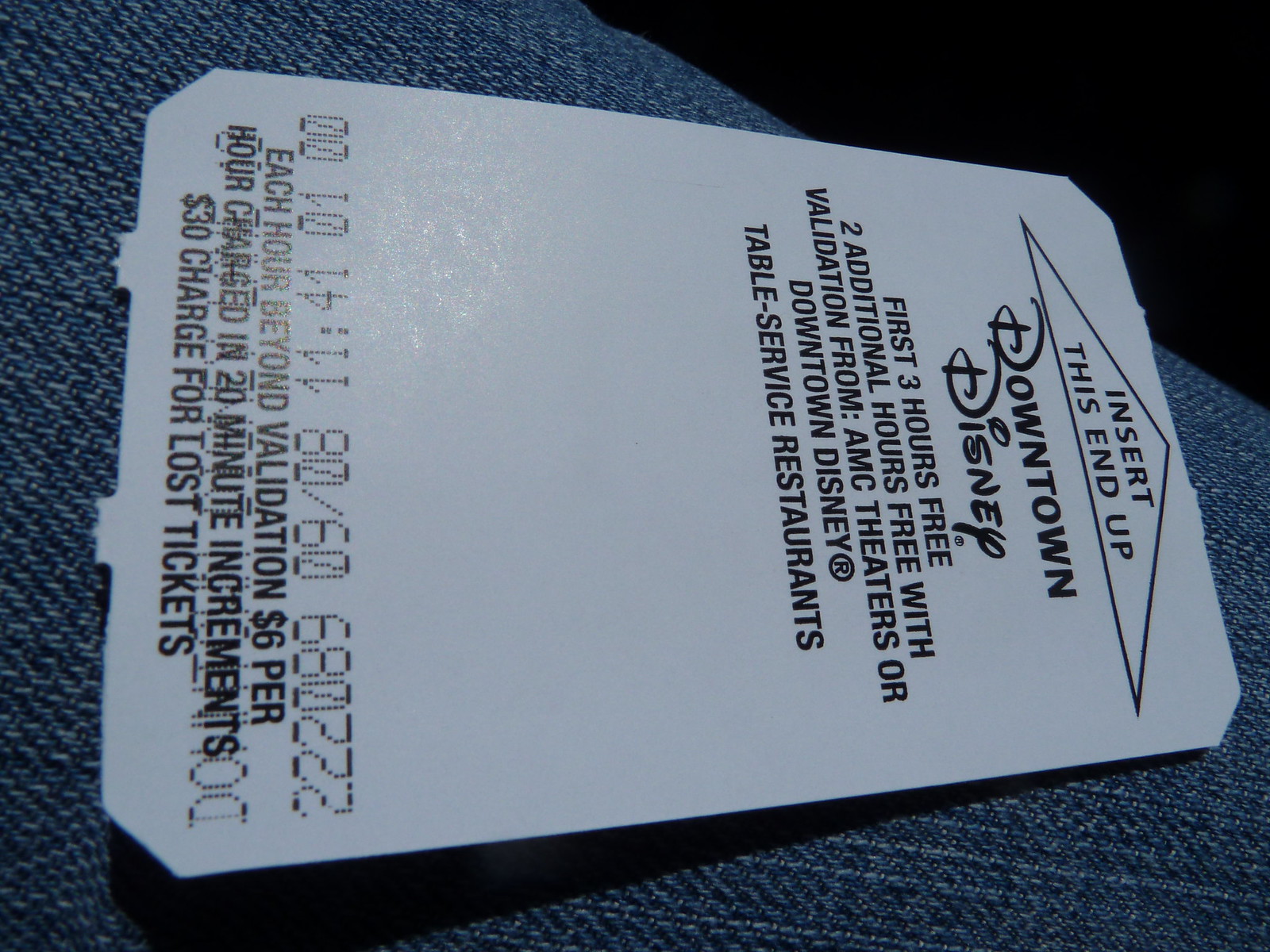The image depicts a close-up of a white, rectangular parking ticket positioned sideways against a blue denim backdrop, likely on someone's jeans. The top of the ticket features an arrow with the instruction "insert this end up," followed by the text "Downtown Disney" in the distinctive Disney font. Below this, it states "first three hours free, two additional hours free with validation from AMC Theaters or Downtown Disney table service restaurants." Further down, the ticket details additional costs: "each hour beyond validation $6 per hour, charged in 20-minute increments" and a "$30 charge for lost tickets." The bottom of the ticket displays a series of numbers, indicating the terms and conditions of the parking fees.